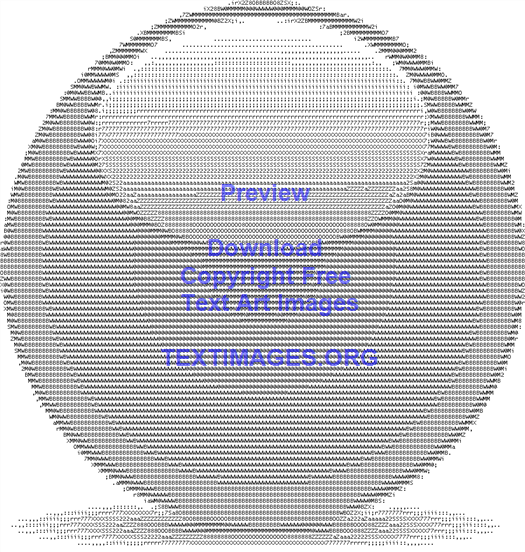This digital artwork showcases an intricately designed bowl composed entirely of small-sized numbers and alphabets rendered in carefully organized patterns. The bowl, primarily built in dark grey hues, features a lighter grey spot at the top, creating an effect akin to a bright spot or hole. The artwork's three-dimensional form is emphasized through the shading, with darker tones on the outside and gradations of lighter grey towards the center. The bowl appears to float above a small shadow-like base, adding depth to the composition. Atop this visual, blue text reads "Preview, Download, Copyright Free, Next Art Images, Text Images.org" against a clean white background, denoting its source and content information. This unique piece strikes a balance between abstract digital creation and typographical art, engaging viewers with its meticulous detail and innovative use of characters.